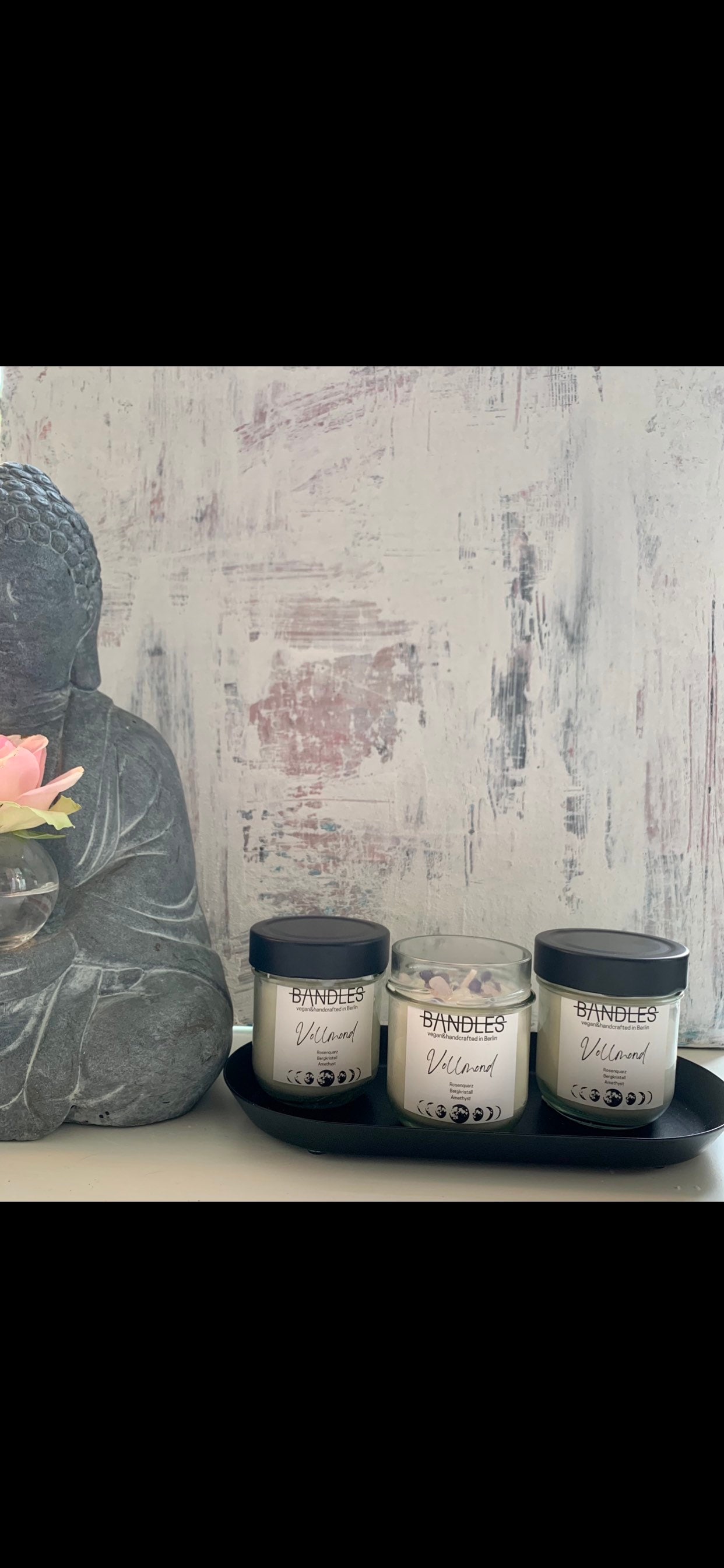The indoor color photograph features a central focus on a black oval platter holding three clear jars with white labels and black text, prominently displaying the brand name "BANDLES" along with an illegible cursive word and a depiction of the moon phases. The jar in the middle is uncapped, revealing crystal-like contents, while the two jars on either side are secured with black lids. Positioned to the left on a beige surface is a gray statue of Buddha, partially cropped by the edge of the image, clutching a glass bowl that contains a pink flower floating in water. The backdrop is a whitewashed wall with visible patches of faded orange and black, adding a rustic feel to the scene. The top and bottom sections of the photograph are framed by thick black bands, creating a striking contrast against the lighter background and the detailed elements on the table.